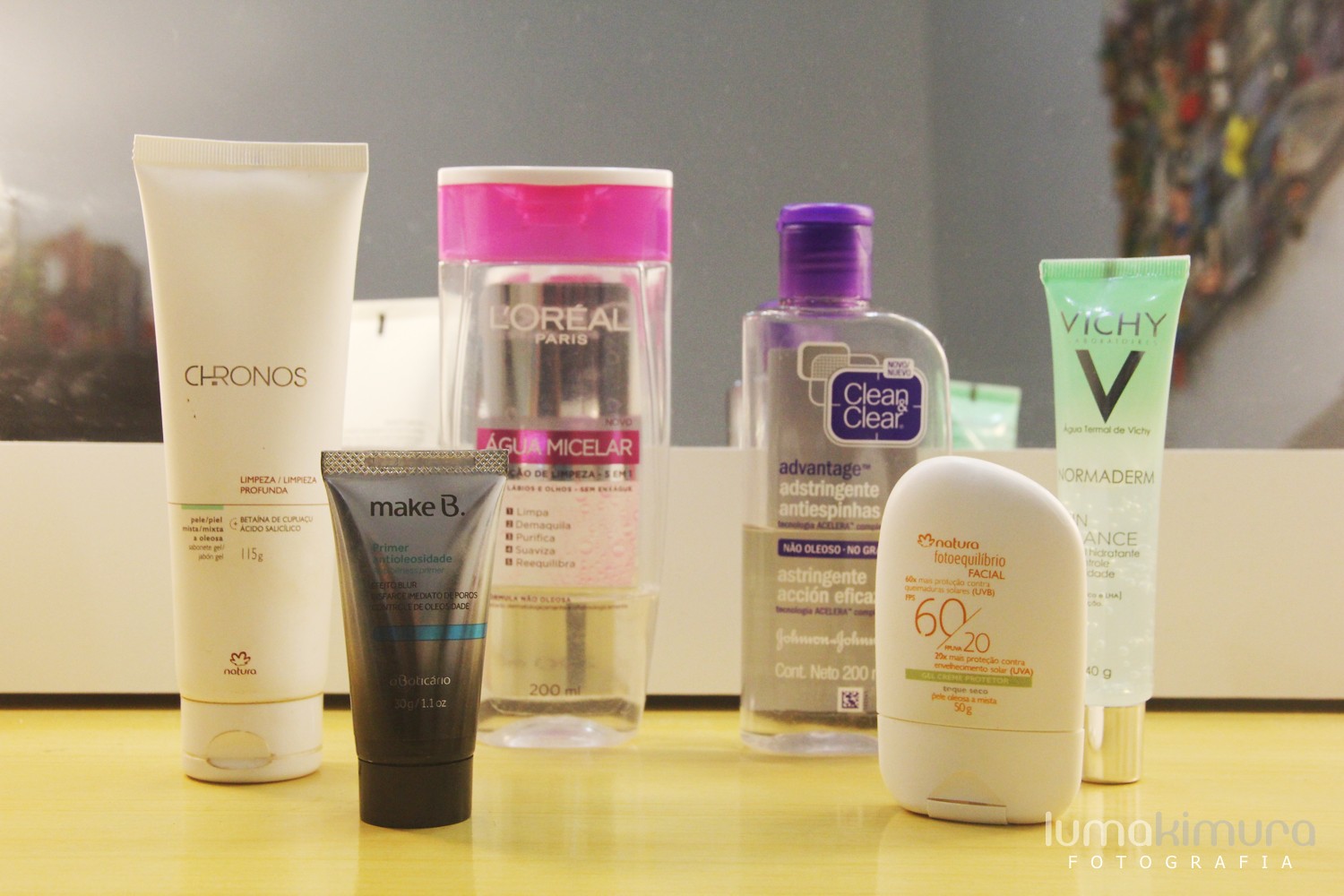This image showcases a collection of cosmetic products and facial cleansers arranged neatly on a vibrant yellow table surface, illuminated by a bright light. A mirror mounted against the wall serves as the backdrop, reflecting the meticulously organized items. In the lower right-hand corner of the image, there is text in varying fonts and colors: "Iyuma" in yellow, "Iyuma Kimura Fotografia" in gray, and additional information in smaller white text.

The table hosts six distinct products, starting from the far left:
1. A white, squeezy lotion bottle with sleek black text stating "Kronos," accompanied by product details in Spanish.
2. Next to it, a smaller, similarly shaped bottle with the name "Make B." The design transitions from a silvery top to black at the base.
3. Behind but adjacent to it, there's a clear container labeled "L'Oreal Paris" with a pink lid.
4. Following this is another clear container with a purple lid, labeled "Clean and Clear."
5. A smaller, egg-shaped container marked "Natura," featuring additional Spanish text.
6. Finally, a product labeled "Vichy," characterized by a mint green gradient and a prominent "V" that transitions into a sparkly gold cap.

The careful arrangement and the varied designs of the containers create a visually appealing display, hinting at a diverse range of skincare solutions.